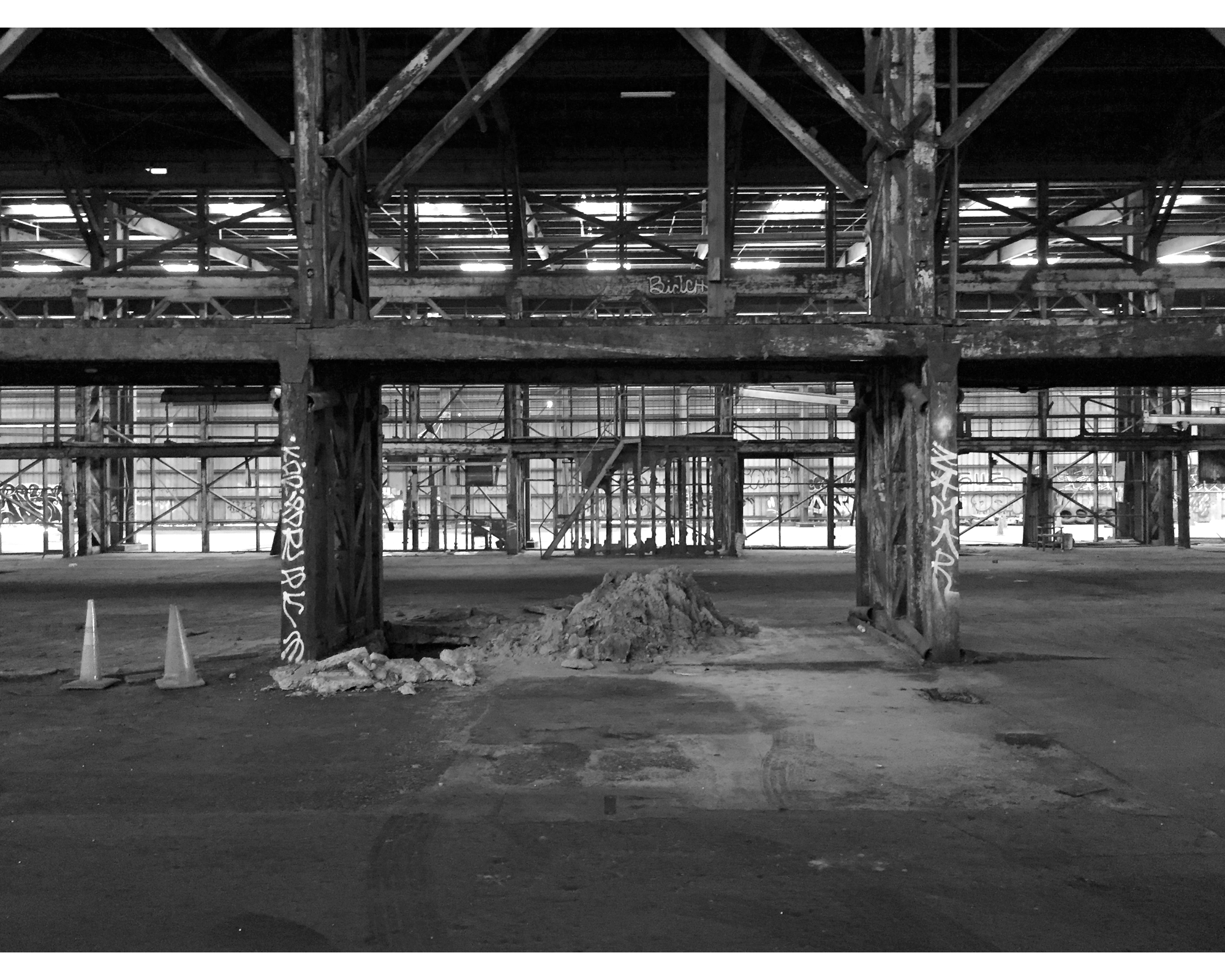This black and white photograph captures an abandoned or under-construction warehouse-like building, now a barren construction site with no walls. The image reveals an intricate lattice of exposed scaffolding and metal beams crisscrossing overhead, creating a dark, industrial atmosphere accentuated by the predominance of dark tones and shadows. Fluorescent lights are mounted on the ceiling, yet the space remains bathed in natural, subdued daylight. At the center of the picture lies a prominent pile of sand or dirt, flanked by two traffic cones on the left side. The cement floor is marked with tire tracks leading to or from this central mound, suggesting recent activity. Although graffiti is scarce within this frame, the visible sections of the interior and distant walls are marked with scattered tags, hinting at neglect and abandonment. The scene outside, glimpsed through the skeletal structure, is heavily adorned with graffiti, accentuating the forsaken vibe of this deteriorating industrial setting.